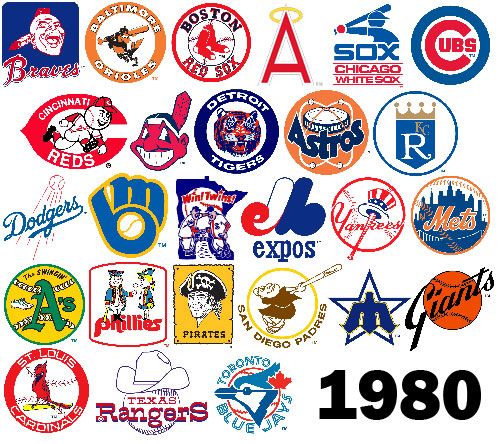The image showcases a grid of MLB team logos from 1980, arranged on a white background. Each logo represents a different team, totaling around 27 logos. The teams include the Boston Red Sox with their classic logo, the Angels featuring a red "A" with a yellow halo, and the Cubs with their iconic red "C" enclosing the word "Cubs." Other highlights include the Dodgers with their blue scripted name, the Cardinals adorned with a red bird, and the Giants with scripted typography. Each row contains about five to six logos, featuring nostalgic symbols such as the Braves' logo with an Asian American figure on a blue field, the Orioles, White Sox, Reds, Indians, Tigers, Astros, Royals, Mets, Twins, Expos, Yankees, A's, Phillies, Pirates, Padres, Rangers, and Blue Jays. Notably, the Astros logo of that era stands out as a significant emblem from that period.